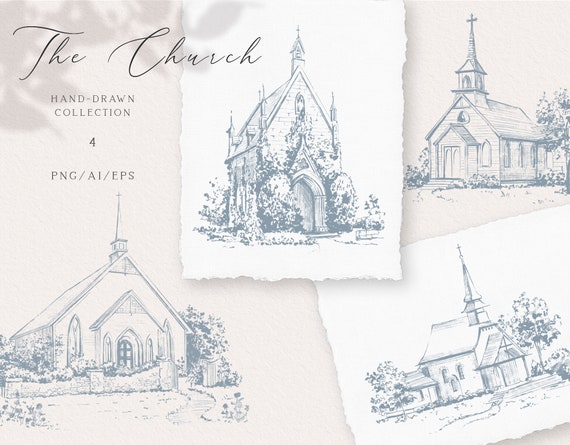This black-and-white photo is a detailed compilation of four hand-drawn church buildings in pencil, ink, or pen, presented on torn bond-like paper. Each church is depicted from a frontal perspective, showcasing a variety of architectural styles. At the top left, in black cursive script, the text reads "The Church," and below it states "Hand-Drawn Collection for PNG-AI-EPS."

- **Top Left Church**: This broad-peaked church features an entrance adorned with a stone-stacked fence, a winding walkway, and stained-glass windows flanking the doors. It boasts a tall steeple with a cross atop.
- **Middle Top Church**: A very narrow and tall structure, this church has spires at its corners and a stone entryway surrounded by plantings and bushes.
- **Bottom Left Church**: With a pointed roof and a secondary pointed structure topped with a cross, this church has arched windows and doors, and is surrounded by some bushes.
- **Bottom Right Church**: This Puritan-style New England church, made of clapboard, is characterized by evenly spaced stained-glass windows and stairs leading up to double front doors. It features a more elaborate entrance with additional connected buildings and a peaked roof with curved sides.

The artwork is distinguished by its grayscale palette, employing shades of gray, white, and charcoal. Each drawing is intricately detailed, capturing the unique characteristics and landscaping around each church.